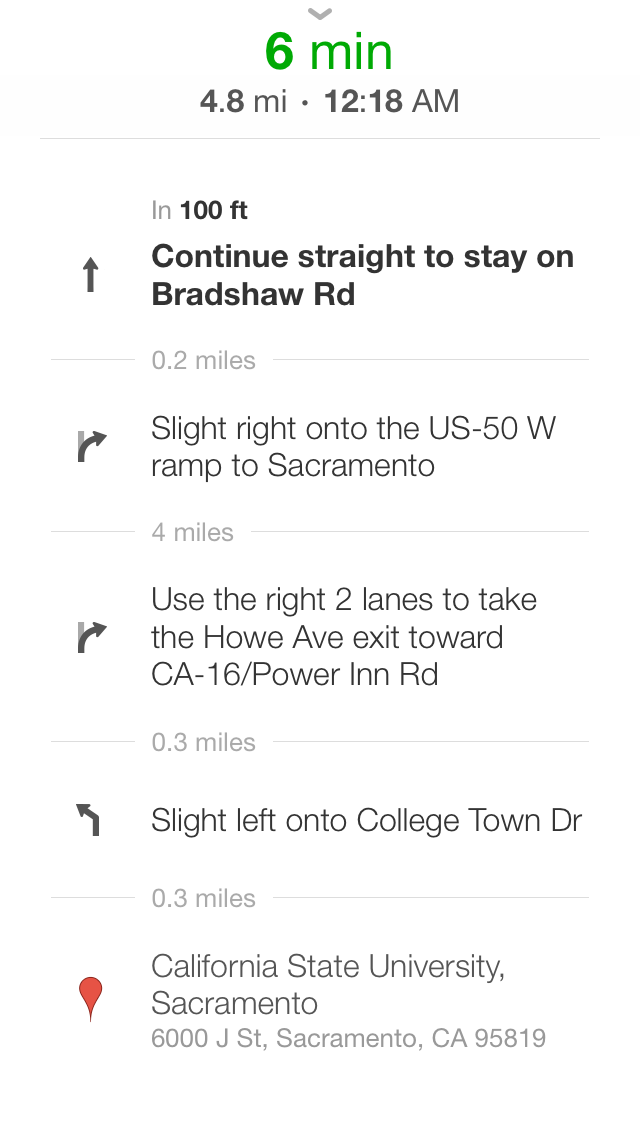The image depicts detailed turn-by-turn directions from a starting location to Bradshaw Road in Sacramento, near California State University. The destination is 4.8 miles away and estimated to be reached in six minutes, with an arrival time of 12:18 AM. The directions are displayed using black Arial font, with arrows showing the required maneuvers at each intersection. The journey begins at a red balloon-shaped marker, symbolizing the starting point. The directions are neatly organized in a column format, with each step separated into individual rows for clarity.